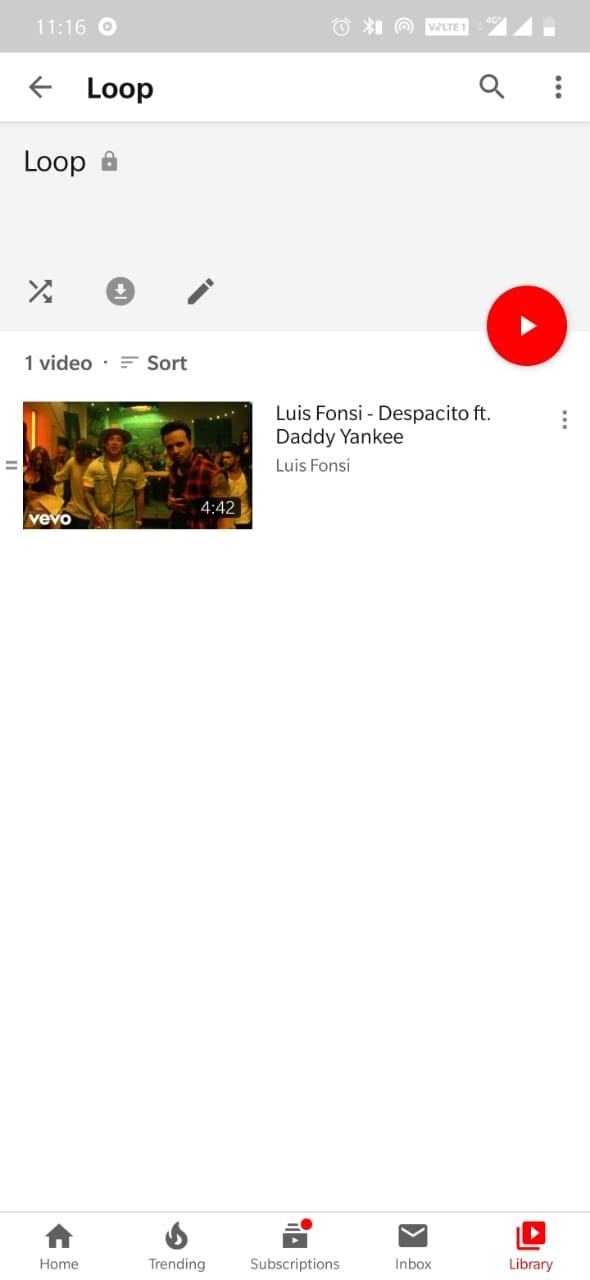This image is a detailed screenshot from a smartphone, capturing the YouTube interface while playing a music video. At the very top, a gray banner displays the status bar with the time, 11:16, along with various phone icons indicating notifications and a battery level at 50%. Below this, there's a white navigation bar featuring a back arrow, loop button, search magnifying glass, and a three-dot menu for additional options. 

Further down, a light gray control bar is visible, providing options for looping the video, sorting, downloading, and editing with corresponding icons. Prominently displayed in the middle of the screen is the video itself, easily identifiable by the red play button with a white triangle in the center and the recognizable Vevo logo in the bottom-right corner.

The content of the video shows two men, one dressed in a cardigan and the other in a plaid shirt, both with dark hair. This snapshot is from the popular music video "Despacito" by Louis Fonsi featuring Daddy Yankee, with a total duration of 4 minutes and 42 seconds.

At the bottom of the screen, the YouTube app's primary navigation tabs are visible: Home, Trending, Subscriptions, Inbox, and Library. This well-captured screenshot summarizes the user interface and specific details of the video being viewed on the phone.